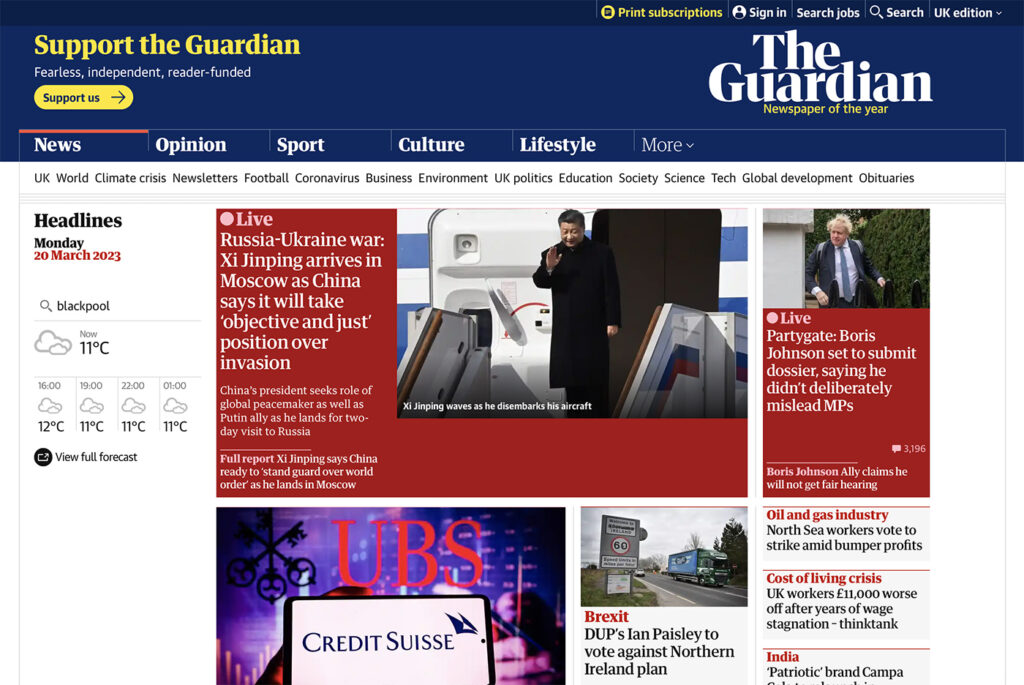Here's a cleaned-up and detailed caption:

---

This image captures the front page of The Guardian newspaper. A prominent blue banner spans across the top, featuring "Support The Guardian" in the upper left corner, accompanied by the phrase "Fearless Independent Leader Funding" and a "Support Us" button. The Guardian's name is prominently displayed in large text on the far right, with "Newspaper of the Year" written just below it. 

Directly beneath the title, a navigation bar includes tabs labeled News, Opinion, Sport, Culture, Lifestyle, and more. The left side of the page details the day's headlines for Monday, 20 March 2023. A search bar contains the term "Blackpool," with an adjacent weather forecast icon showing a cloud and indicating the current temperature as 11°C. The forecast for different hours of the day is also visible.

The primary headline reads: "Live: Russia-Ukraine War. Xi Jinping arrives in Moscow as China says it will take objective and just position over invasion." To the right, there is a photo of an Asian man standing just outside an airplane door, presumably Xi Jinping.

Below and to the right is another significant headline: "Partygate: Boris Johnson set to submit dossier saying he didn't deliberately mislead MPs," accompanied by an image of Boris Johnson.

Additional headlines outlined include: "DUP's Ian Paisley to vote against Northern Ireland plan," "North Sea workers vote to strike amid bumper profits," and "UK workers £11,000 worse off after years of wage stagnation" attributed to a Think Tank.

---